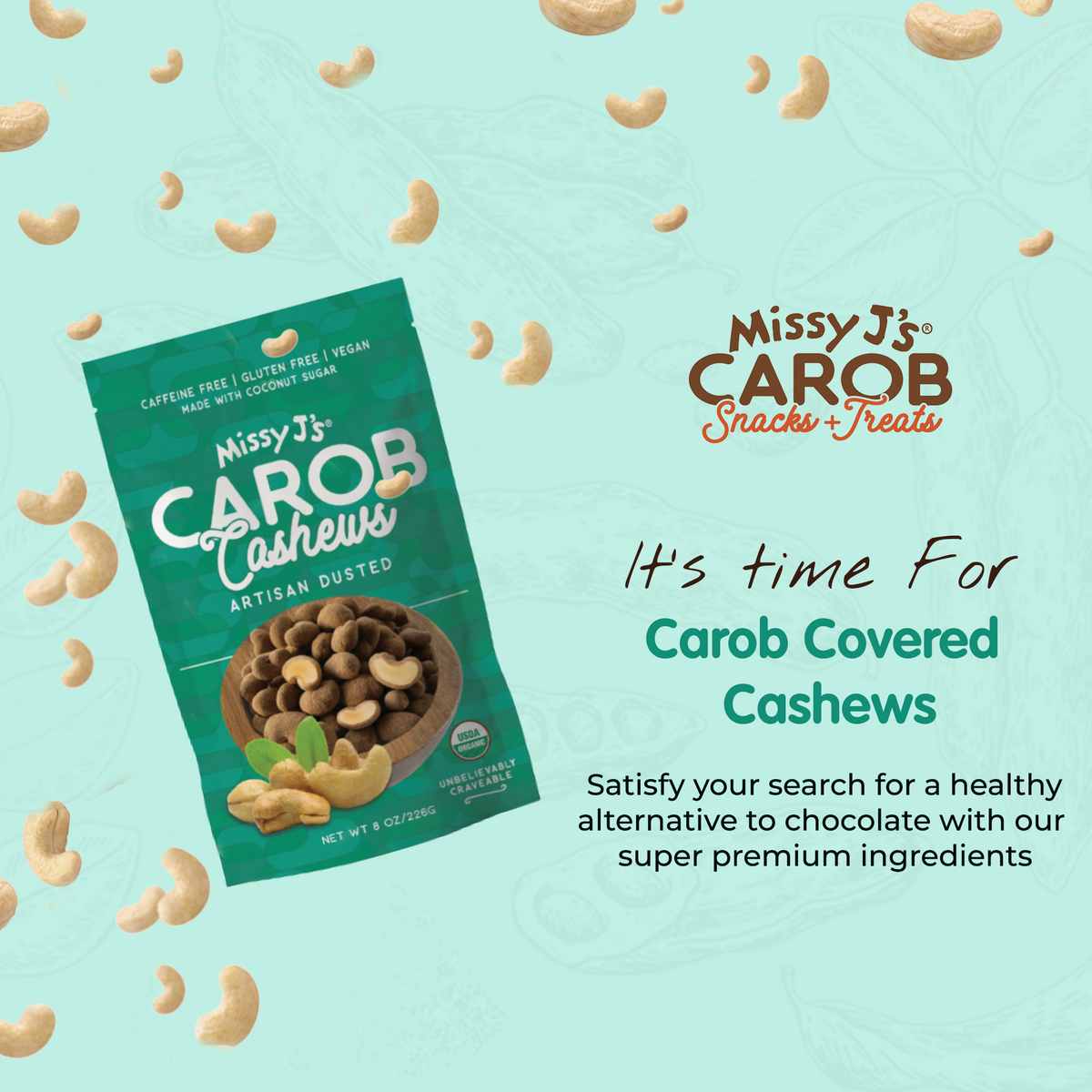The image is a portrait-oriented flyer for Missy J's Carob Cashews, designed with a busy, detailed layout. The background of the flyer is light mint or turquoise with a subtle plant pattern, creating a fresh, natural feel. The left side features an image of the product packaging, which is dark teal with an oval base design. At the top of the package, "Missy J’s Carob Cashews – Artisan Dusted" is written in large white letters, with smaller text above stating the product is "Caffeine Free, Gluten Free, Vegan, Made with Coconut Sugar." The packaging also displays the USDA Organic logo and the net weight of "8 ounces, 226 grams," along with the claim, "Unbelievably Craveable."

On the right side of the image, various fonts highlight key product details. "Missy J's Carob" is written in brown letters, and "Snacks + Treats" appears below in red cursive. "It's time for Carob Covered Cashews" is displayed in a dark teal font, followed by "Satisfy your search for a healthy alternative to chocolate with our super premium ingredients" in a smaller black handwritten font. 

The flyer also showcases a wooden bowl filled with the carob-covered cashews, with some of the cashews cut in half to reveal the coating. Cashews appear to be falling from the sky, adding a whimsical touch to the advertisement. Overall, the image conveys a busy yet inviting presentation of a healthy, vegan snack alternative.